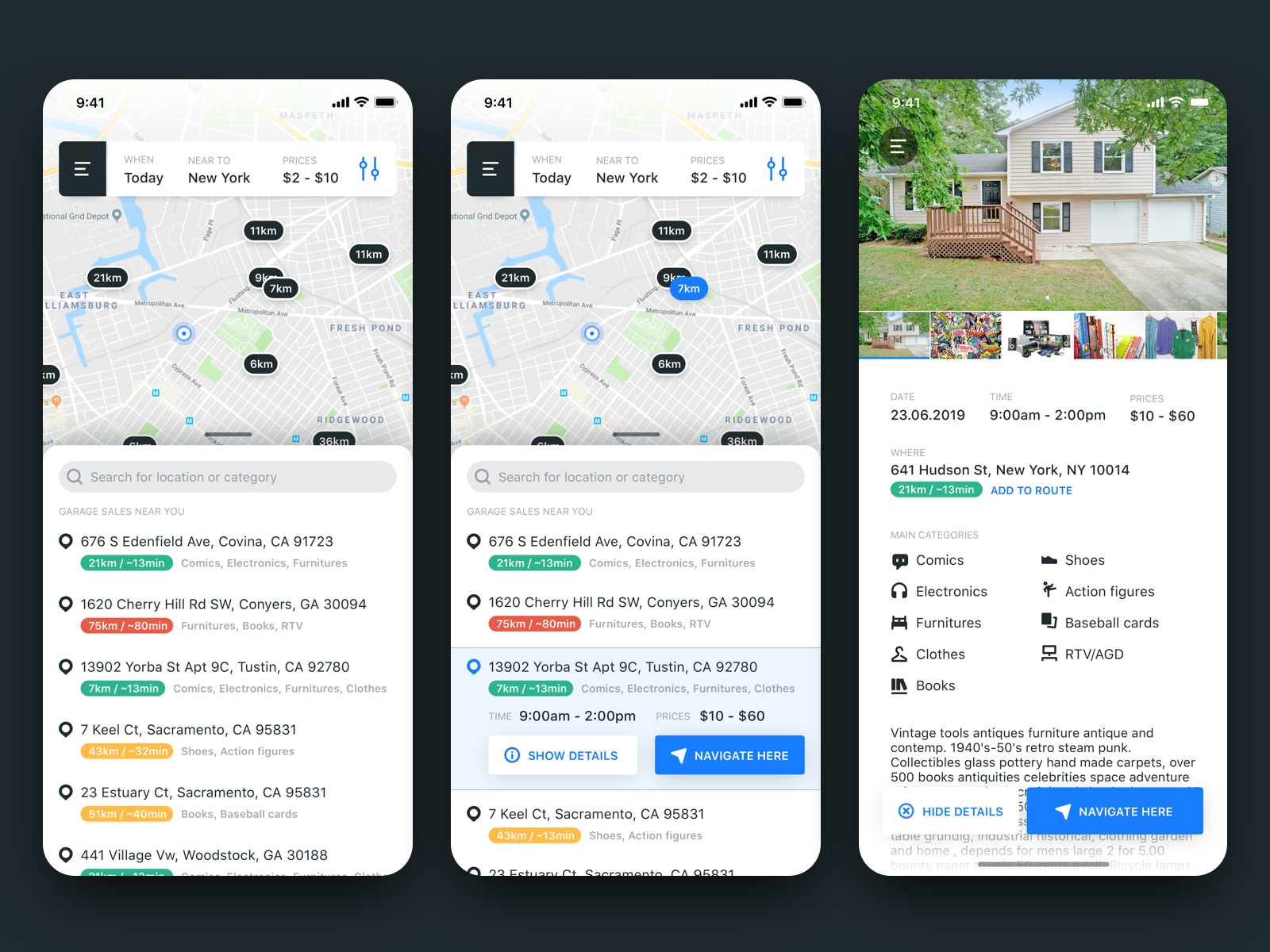The image is set against a black background and features three screenshots from a mobile phone. Each screenshot provides detailed information about various garage sales in different locations.

1. The first screenshot:
   - Displays the current time as 9:41.
   - Mentions "when today near to New York" with prices ranging from $2 to $10.
   - Shows a map with distance markers for various locations.
   - Lists multiple garage sale locations with distances and estimated travel times:
     - **676 South Edenfield Avenue, Covina, California 91723:** 21 kilometers, 13 minutes. Items: Comics, electronics, furniture.
     - **1620 Cherry Hill Road Southwest, Conyers, Georgia 30094:** 75 kilometers, 80 minutes. Items: Furniture, books, RTV.
     - **13902 Yorba Street, Apartment 9C, Tustin, California 92780:** 7 kilometers, 13 minutes. Items: Comics, electronics, furniture, clothes.
     - **7 Keele Street 7 Keele Court, Sacramento, California 95831:** 43 kilometers, 32 minutes. Items: Action figures.
     - **23 Estuary Court, Sacramento, California 95831:** 51 kilometers, 40 minutes. Items: Books, baseball cards.
     - **441 Village VW Woodstock, Georgia 30188:** (mostly cut-off).

2. The second screenshot:
   - Similar "when today near to New York" heading with prices $2 to $10.
   - Displays the same map with marked areas.
   - Lists the same addresses but highlights **13902 Yorba Street, Apartment 9C, Tustin, California 92780:**
     - Distance: 7 kilometers, 13 minutes.
     - Items: Comics, electronics, furniture, clothes.
     - Time: 9 a.m. to 2 p.m.
     - Prices: $10 to $60.
     - Options: Show details, Navigate here.

3. The third screenshot:
   - Shows an image of a two-story white house with two small garage doors, wooden steps, and railing leading to the front door.
   - A patchy green lawn and a white driveway with no cars parked.
   - Detailed information:
     - Date: June 23, 2019
     - Time: 9 a.m. to 2 p.m.
     - Prices: $10 to $60.
     - Location: 641 Hudson Street, New York, NY 10014
     - Distance: 21 kilometers, 13 minutes.
     - Options: Add to route, Hide details, Navigate here.
   - Lists main categories available at the garage sale, including:
     - Comics, shoes, electronics, action figures, furniture, baseball cards, clothes, RTV/AGD, books, vintage tools, antiques, 1940s-50s retro, steampunk, collectibles, glass, pottery, handmade carpets, over 500 books, antiquities, celebrities, space, adventure.
   - Part of the text is obscured by two rectangles:
     - White rectangle: "Hide details" in blue lettering.
     - Dark blue rectangle: "Navigate here" in white writing.